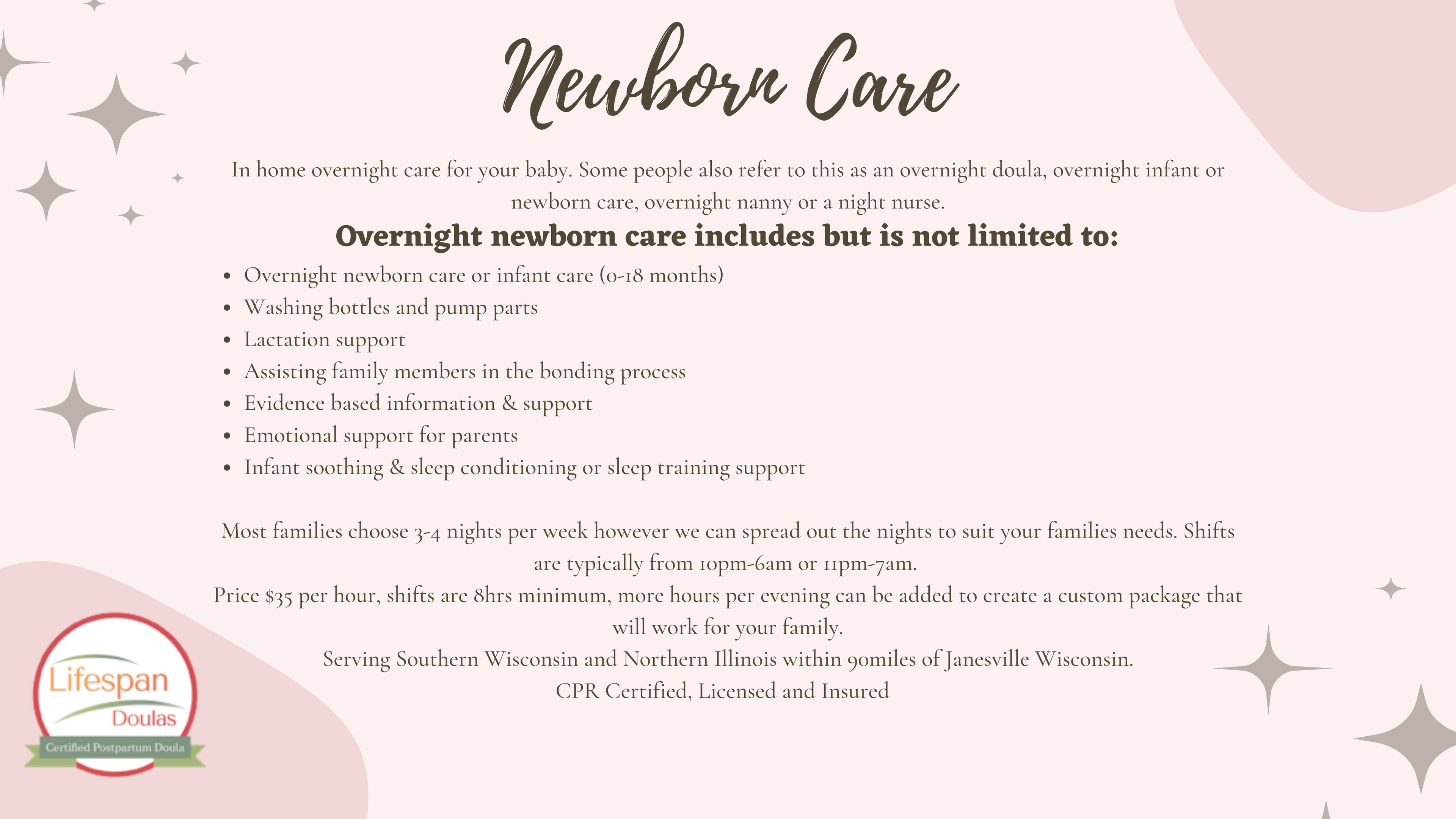The image is a detailed and decorative piece, possibly taken from a magazine, brochure, postcard, or seminar presentation, providing extensive information on newborn care. Dominated by text, the top of the image features the heading "Newborn Care" in large, prominent script, adorned with decorative stars on the top left and bottom right. The content focuses on in-home, overnight care services for newborns, also referred to as overnight doula or night nurse services. The list under the heading outlines various aspects of overnight newborn care, including caring for infants aged 0 to 18 months, washing bottles and pump parts, offering lactation support, and assisting family members in bonding with the newborn. This informative piece appears to market superior care services, potentially offered by a hospital or at a seminar/webinar aimed at new or expecting parents seeking specialized newborn care.